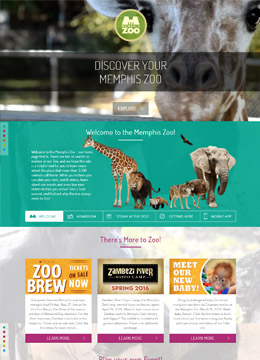This image is a depiction of the homepage or discover page for the Memphis Zoo. The layout is divided into three distinct sections:

1. **Top Section**: This portion features a slightly low-resolution background image that includes a close-up of a giraffe's face on the right side, with blurred greenery and possibly a fence on the left. Overlaying this background is a circular button and a prompt to start navigating the content. At the bottom of this top section, there's a transparent, horizontal rectangle with more navigational or informational text.

2. **Middle Section**: Dominated by a teal background, this segment has a welcoming message— "Welcome to the Memphis Zoo" in white text prominently positioned at the top. Additional white text is placed towards the left side, possibly serving as headings or brief descriptions. The bottom of this section includes five selectable boxes, likely representing different animal categories or zoo highlights. The first box on the left is currently highlighted. To the right side of this section is an image collage featuring various zoo animals, taking up more than half of the right side of the image. The animals depicted include a giraffe, lion, red panda, wolf, ostrich, and an elephant. There’s also an image of a bird in flight near the elephant.

3. **Bottom Section**: This area showcases three advertisement banners for upcoming zoo events against the existing background, reinforcing ongoing or future attractions.

Overall, the homepage is vibrant and visually engaging, designed to captivate visitors with glimpses of zoo highlights and essential information about the Memphis Zoo.